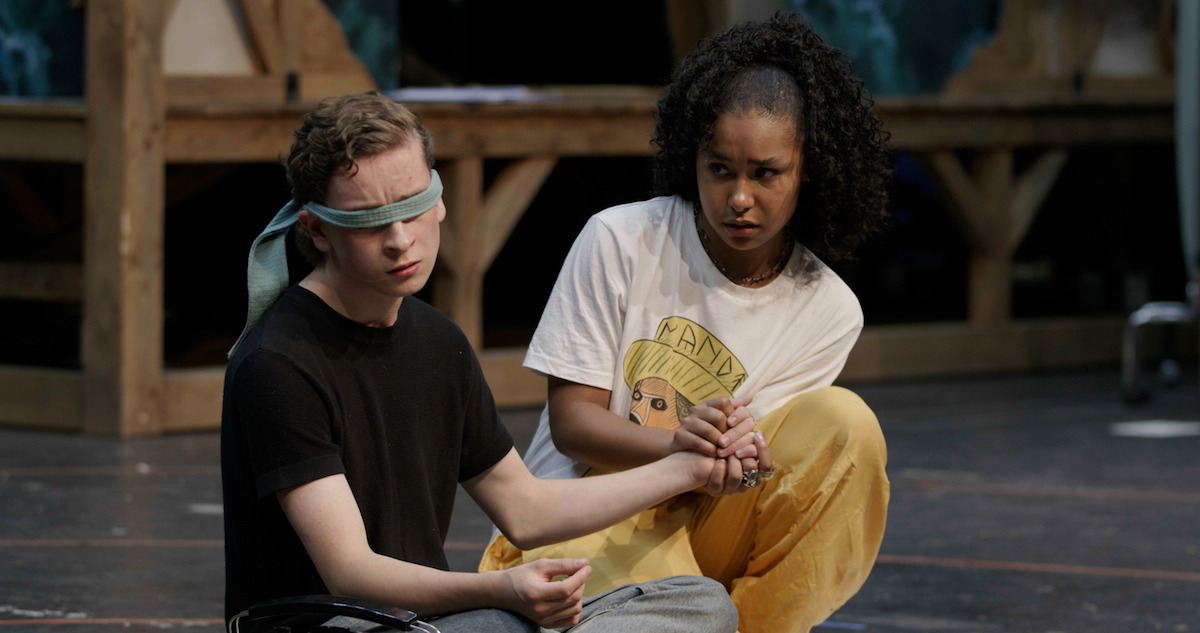The photo captures a poignant moment between two children seated on a cement floor. The girl, with long black hair, dons yellow pants and a white T-shirt featuring a figure in a hat. She is tenderly holding the hand of a younger boy to her left. The boy, dressed in a black T-shirt, wears a blue-green blindfold reminiscent of a necktie or bandana, which partially obscures his sad expression. Intricately detailed wood fencing or framing forms the backdrop of this intimate scene, adding a layer of rustic charm with its open design supported by vertical bars. The girl's two rings add a subtle touch of individuality to this emotionally resonant image.